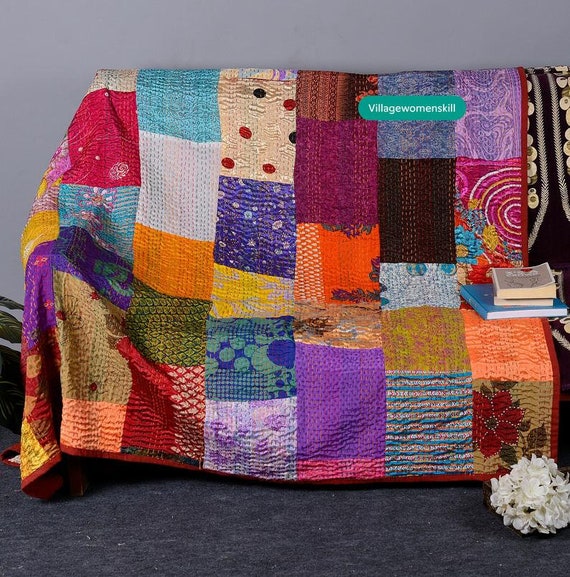In the center of this indoor photograph is a couch or futon draped with a vibrant and colorful patchwork quilt. The quilt is a kaleidoscope of large rectangles in a variety of bright colors including blue, orange, red, yellow, and purple. Some rectangles feature intricate patterns such as florals, with one notable rose pattern in the bottom right corner. The quilt is laid out so that it covers the couch entirely from the floor to the backrest.

On the right side of the couch, atop the quilt, lies a small stack of three books: the bottom one is a blue hardcover, with two paperbacks stacked above it. On the floor in front of the couch, near the books, is a bouquet of white flowers. The scene is set against a backdrop of a gray wall and a gray, possibly blue, short-pile carpet. To the left of the couch, partially visible, are a few green leaves from a houseplant. Additionally, the quilt features a green rectangle with white text that reads "Village Women's Kill" at the top. The entire setup of the photograph brings out the intricate beauty of the quilt against the neutral tones of the room.